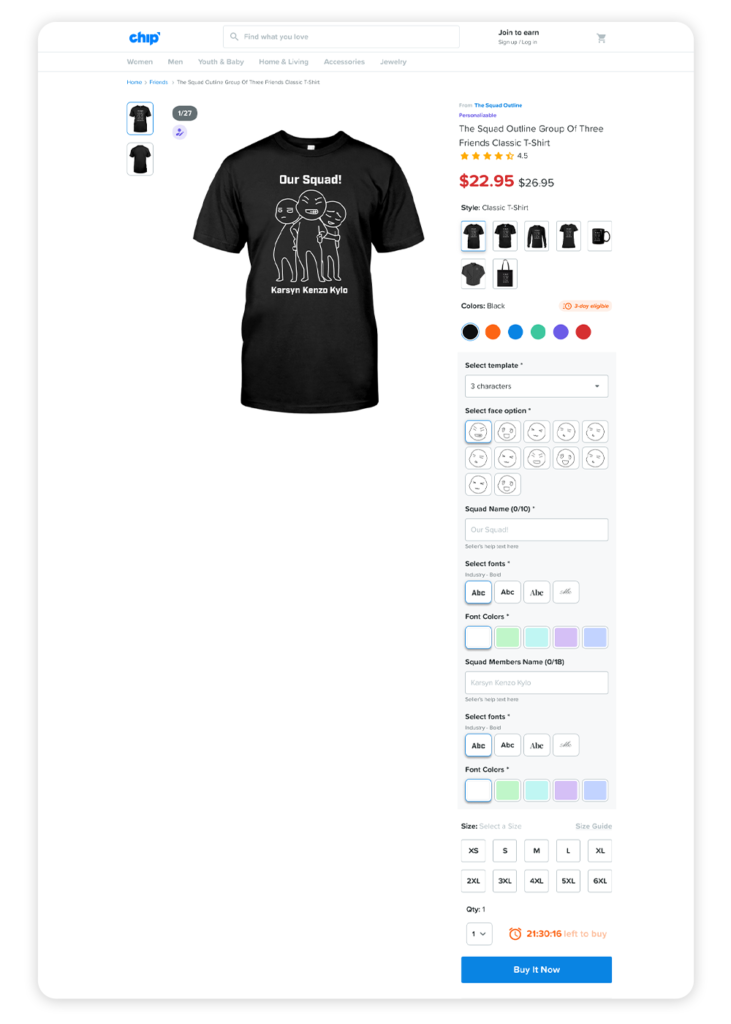This screenshot depicts a web page with a predominantly white background, displaying a product listing for a black t-shirt. In the top left corner of the page, the word "chip" is written in blue letters. Due to the low resolution, the image appears somewhat grainy and blurred in specific areas.

At the top of the page, a gray search bar is prominently placed with the prompt "Find what you love and join to earn." To the right of the search bar, there are buttons labeled "Sign Up" and "Login." Below this, a horizontal navigation menu displays categories including "Women," "Men," "Youth and Baby," "Home and Living," "Accessories," and "Jewelry."

The main focus is on a black t-shirt with a simplistic, yet engaging design. The shirt has "Our Squad" printed in white letters and features a minimalist illustration of three figures labeled Carson, Kenzo, and Kylo. On the right side of the image, a product description is provided: "The Squad Outline Group of Three Friends Classic T-Shirt." Customer reviews rate the shirt at 4.5 stars out of 5.

Retailing for $22.95, the t-shirt is showcased through several images displaying different angles. The product page also offers variations, such as a classic long t-shirt, along with an assortment of additional merchandise, including cups and bags. The selected color for the t-shirt is black, but other available colors include orange, blue, green, and red. There is also an option to customize the characters' faces depicted on the shirt.